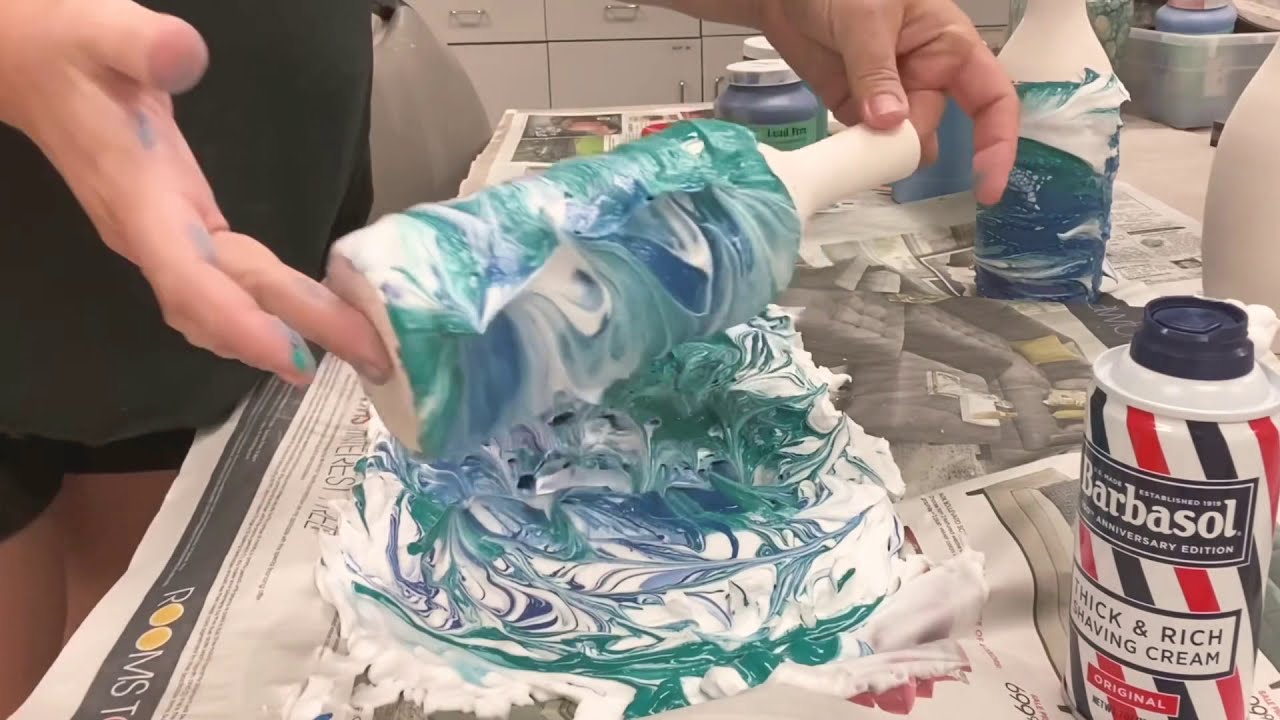In this photograph, a person, predominantly visible from the upper left corner, is engaged in an unusual craft project. Wearing a black shirt and black shorts, they’re handling a rolling pin coated in a mixture of green, blue, and white substances. It appears they are using Barbasol shaving cream, evident from the can with its distinctive white, red, and blue diagonal stripes prominently placed on the table. The individual is applying the cream-turned-faux frosting to a round object that mimics the shape of a cake atop a table covered with newspaper. The scene is set in what looks like a classroom, suggested by the background clutter of paint tubs, another roller, and shelves or cubbies, indicating an arts and crafts session that might be producing this bizarre, non-edible creation. The hands of the person, spotting traces of the creamy mixture, work deftly in this creative yet somewhat surreal endeavor.